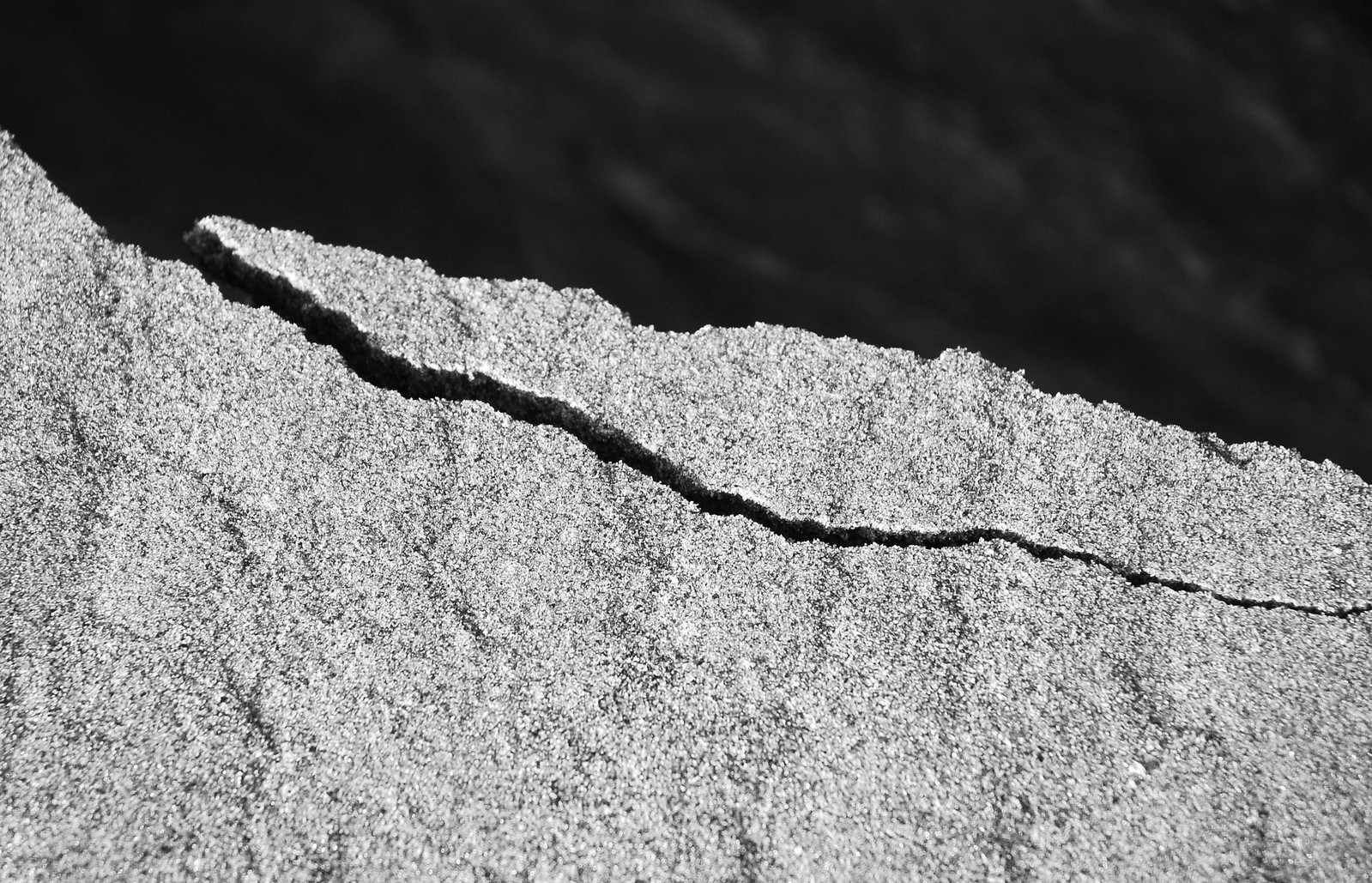A horizontally aligned rectangular photograph captures a rough-textured granite-like rock surface with a striking rugged edge. Dominated by shades of grey, white, and black, the rock features a prominent crack running from the top left corner to the bottom right corner. The fissure is wider on the upper left side and narrows as it descends to the bottom right. This indicates an impending break, with a significant chunk of rock poised to detach from the cliffside and plummet into the body of water below, which is implied by the dark, slightly blurry area at the top of the image. The lighting throughout the photo strongly suggests it was taken during the daytime. The rock's grainy, rough surface and the large, impending crack create a dramatic portrayal of nature's erosion process.